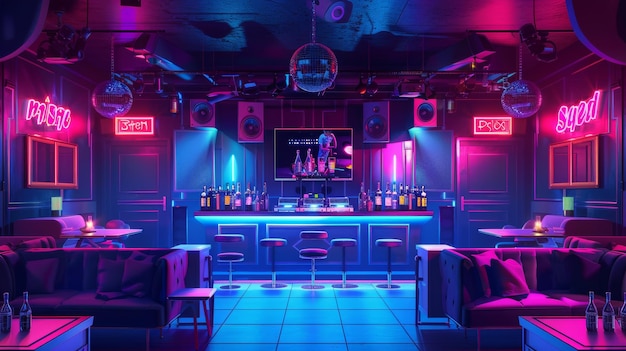This image showcases a futuristic, AI-generated bar bathed in neon lighting. Dominating the center is a sleek bar counter surrounded by stools, with vibrant blue lighting underneath and pink neon hues enveloping the surroundings. Three disco balls hang from the ceiling, casting reflections around the space. On the left and right of the bar are lounge areas furnished with large couches, pillows, tables, and booths. The neon signs scattered throughout, although bright and vivid, contain characters or symbols that do not form coherent words, possibly hinting at an abstract or foreign script. Bottles of alcohol are visibly placed on the bar and some tables, adding to the authenticity of the bar setting despite its surreal, AI-crafted ambiance. Mirrors and sporadically placed speakers adorn the walls, contributing to the high-tech, vibrant atmosphere.